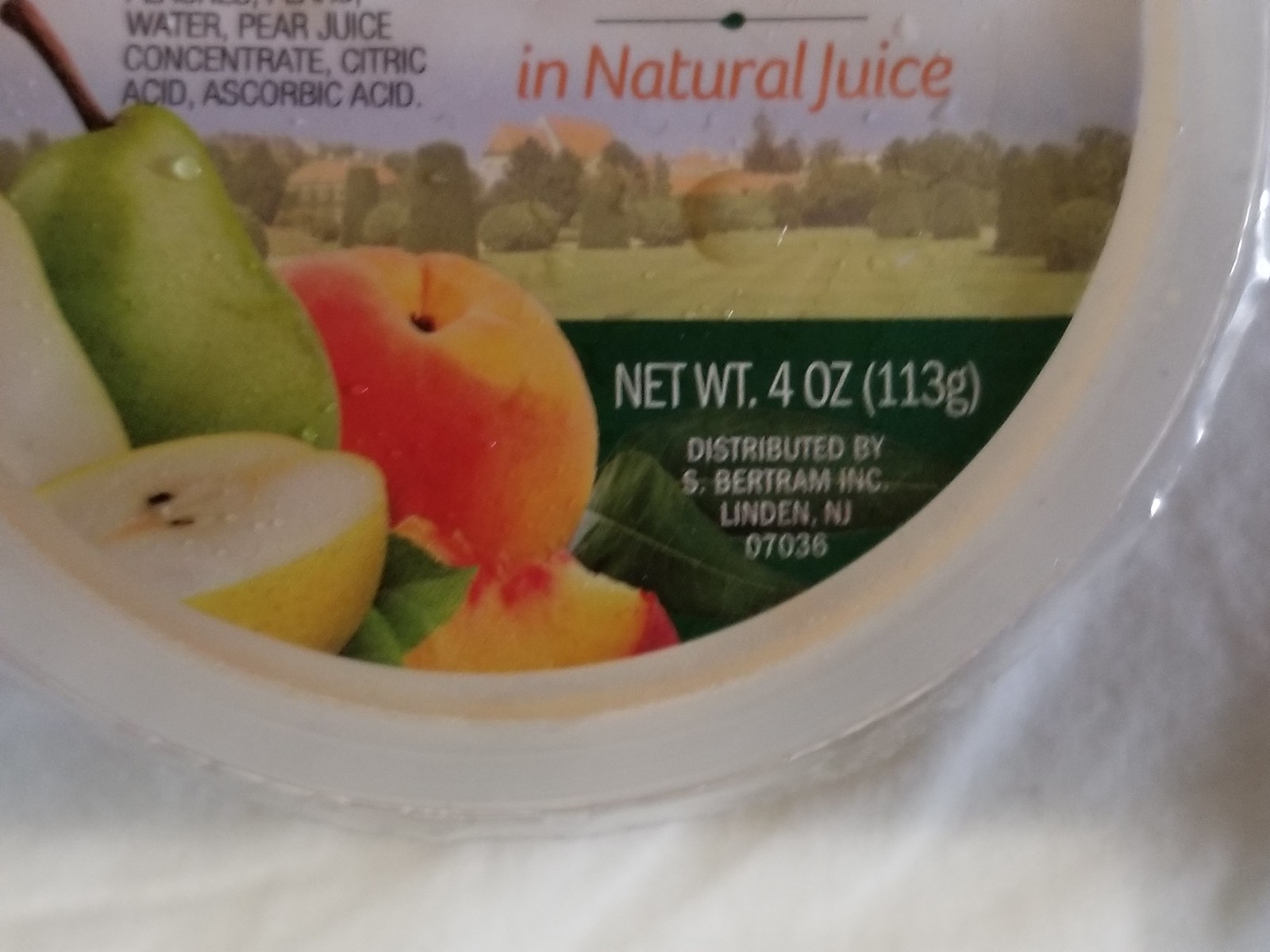The image shows the top of a round food container, likely holding fruit cocktail, set against a white fabric background. The visible portion of the colorful label features various fruits including a green pear and an orangish peach, along with other possible fruits like a yellow or greenish apple. The label text is in both black and orange fonts. Prominently, it reads "water, pear juice concentrate, citric acid, ascorbic acid," and "in natural juice." Additionally, "net weight four ounces (113 grams)" and "distributed by S. Bertram Inc., Linden, New Jersey 07036" are printed in white font. Some parts of the container's label are cut off, making full identification challenging, but it is clear that the product contains fruit in natural juice.